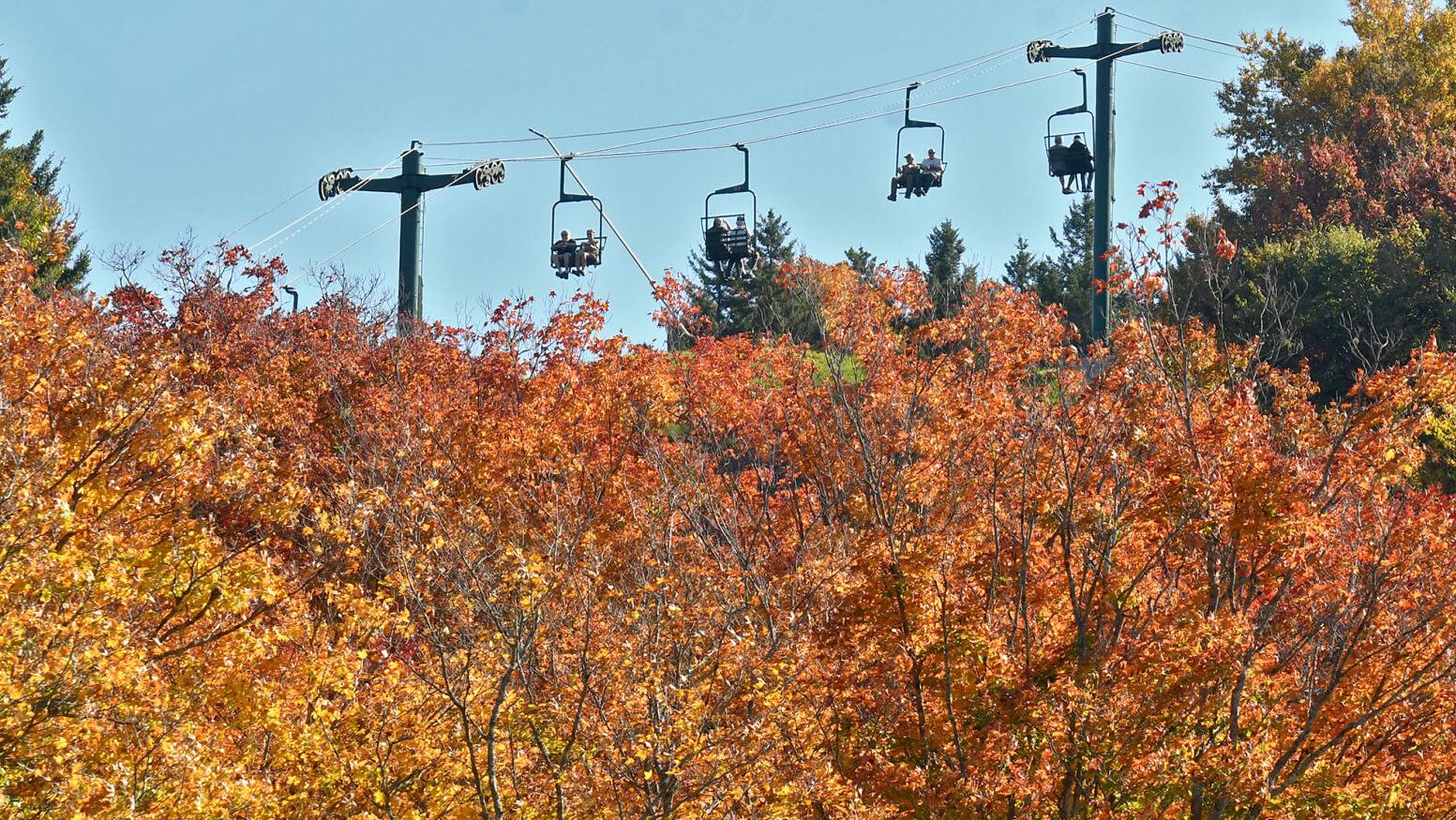The photograph captures the essence of late fall with vibrant foliage, showcasing both burnt orange and yellow leaves in the bottom half of the frame. Among the plants with their autumn colors, there are green trees that add contrast. In the background, against a clear light blue sky, a gondola lift with four two-seater chairs is seen; each chair is occupied by two people. Two of the gondola chairs are heading to the right and two to the left, evoking memories of rides such as those in Gatlinburg, North Carolina. The serene, vivid scene beautifully encapsulates the splendor of fall, highlighting the changing leaves and the peaceful motion of the gondola against the sky.